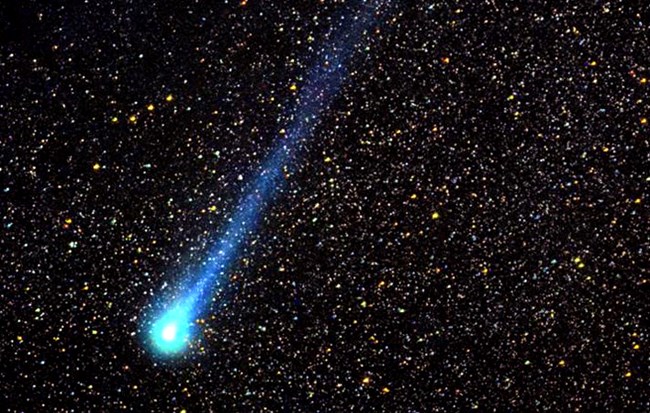This landscape-oriented space photograph captures the Comet Swiss Tuttle amid the meteor shower in the Perseid cluster. The backdrop is a vast, black expanse speckled densely with clusters of white and yellow stars of varying sizes and intensities, creating a richly textured star field. Traversing this dark canvas, a comet or shooting star appears from the top center, moving toward the bottom left corner. The comet features a luminous round center glowing bright blue with a striking white dot in its core. Trailing behind, a light blue tail grows brighter and more vibrant as it extends downward. This detailed space photography image splendidly showcases the comet's radiant path through the densely packed starry night.